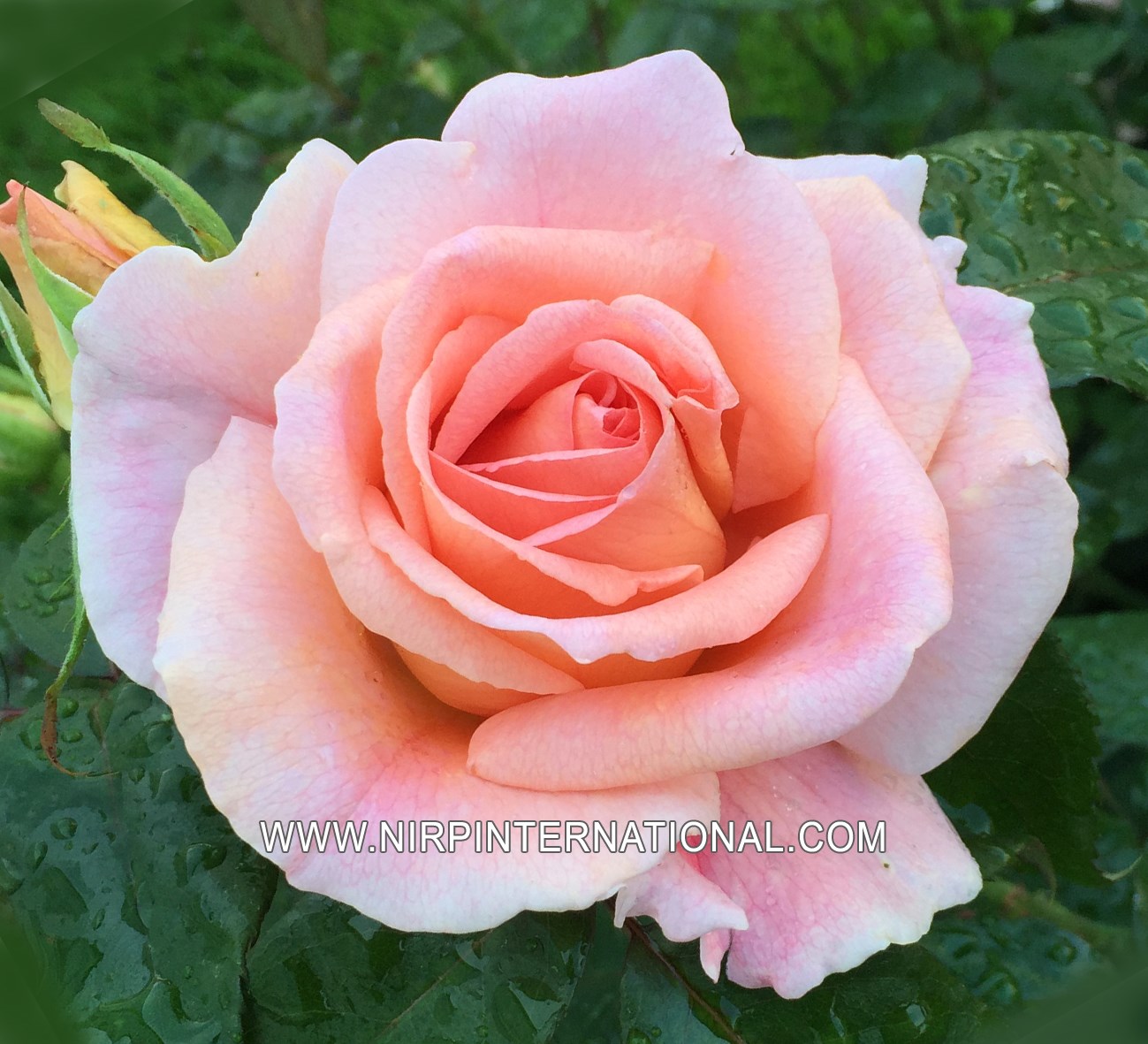This close-up photograph captures a stunning pink rose set in a garden. The rose features petals that intensify in pink towards the center, gradually transitioning to white at the tips. Dark pink veins intricately embellish each petal. The flower appears nearly flawless, with a single small brown dot on one of its lower petals. Surrounding the rose are green leaves, glistening with water droplets as if it just rained, contributing to the fresh and vibrant atmosphere of the scene. In the top left corner, the image displays a budding rose with pink inner petals and yellow outer petals. The slightly blurry background reveals additional greenery, enhancing the garden setting. Over the photograph, there is a caption in white text with a black border that reads "www.nripinternational.com."